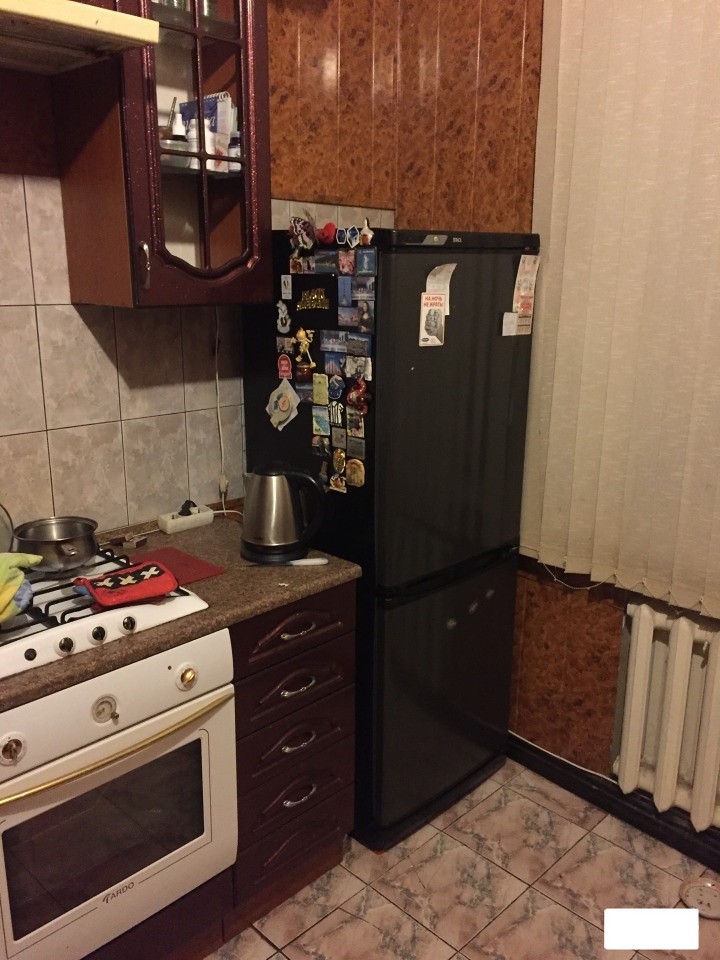This is a detailed portrait-oriented snapshot of a kitchen interior taken from a higher angle, possibly from someone standing on a table. From this vantage point, the linoleum-tiled floor, patterned to resemble faux marble, is prominently visible with some tiles curling at the edges. In the lower right section, a white radiator is mounted to the wall, partially covered by vertical louvered blinds.

To the left of the radiator, a significant feature is the black refrigerator with French doors on top and a bottom drawer freezer. The fridge door exhibits a few pamphlets while its side is densely adorned with a diverse array of magnets and postcards.

Above the fridge are cabinets with a peculiar leathery texture, and to the left side, there's another wall-mounted cabinet with a glass front, cluttered with various items. Below these cabinets, the backsplash is tiled in a square gray pattern.

The countertop along this wall appears to be a solid surface with an integrated stovetop and an oven below, both in white. A base cabinet beneath this area features four dark brown drawers. The stovetop has a pair of oven gloves and some cooking utensils resting on it. Additionally, an area above the stovetop seems designed for an extractor fan, though it's not clearly visible in the image.

In the bottom right corner of the photo, a watermark is obscured by a white rectangle.